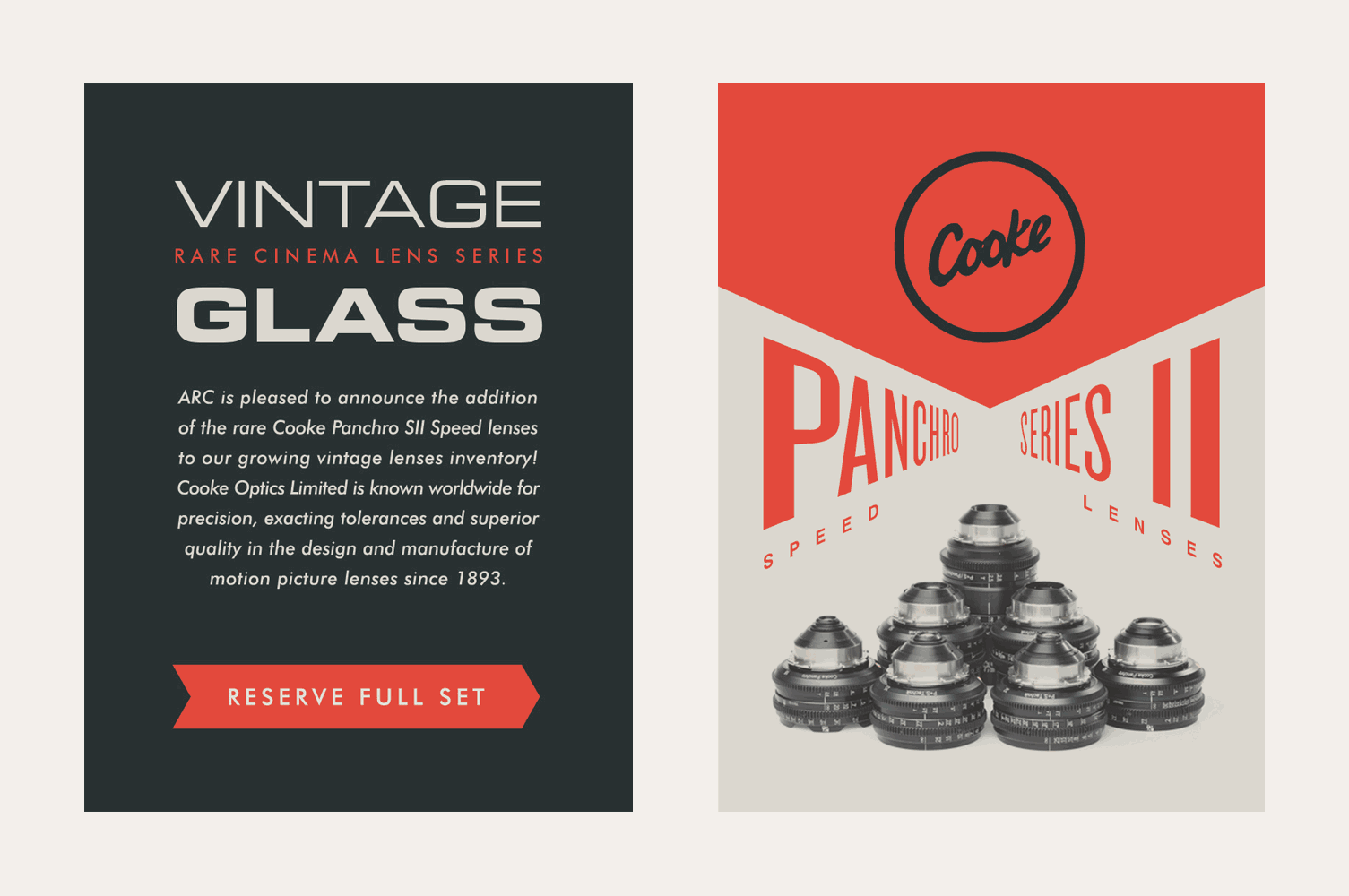This rectangular image appears to be a part of a web advertisement focusing on the promotion of cinema lenses. The left side of the image features a black background with white and red text, introducing the Vintage Glass Rare Cinema Lens Series. It states, "ARC is pleased to announce the addition of the rare Cooke Panchro SII Speed Lenses to our growing vintage lenses inventory." Cooke Optics Limited, renowned globally since 1893 for their precision, exacting tolerances, and superior quality in motion picture lens design and manufacture, is prominently mentioned. Beneath this information, a red arrow with the text "Reserve Full Set" points to the right, adding a call-to-action element. 

On the right side of the image, a stack of about seven cinema lenses is arranged in a pyramid form. The top portion of this section features a black circle with the word "Cooke" inscribed in cursive. Above the lenses, there's a red triangle pointing downwards with the text "Panchro Series II Speed Lenses," reaffirming the product's identity. This meticulous layout combining the advertisement's dual nature effectively highlights the product while maintaining brand consistency.